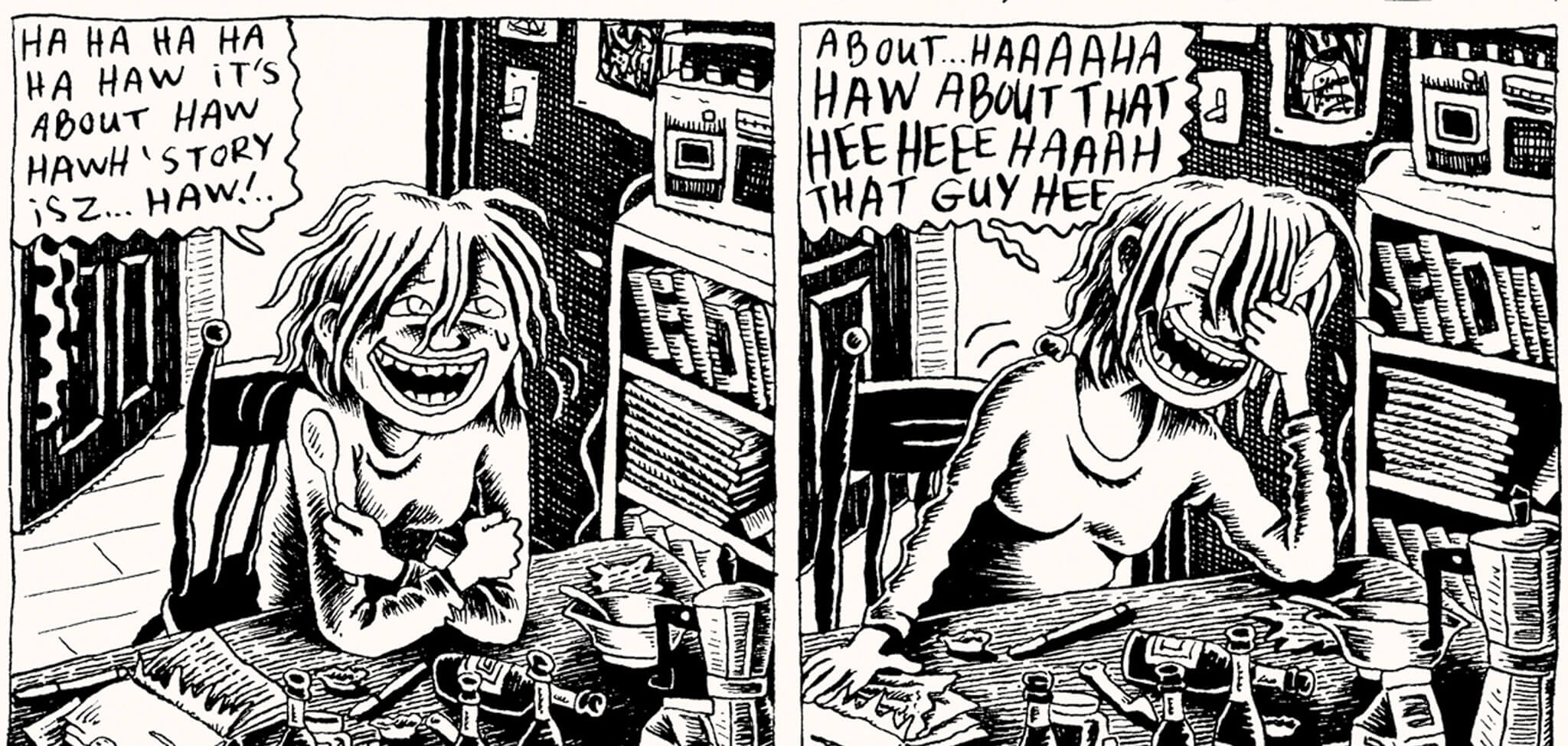The image is a black-and-white, landscape-oriented comic strip consisting of two square panels side-by-side. Both panels depict the same scene: a woman with chin-length, frazzled hair sitting at a cluttered table filled with various items like bottles and a book with a ripped page. A spoon is held in her hand in both illustrations. 

In the first panel, the woman is leaning on her elbows, looking up with a wide, maniacal grin, and tears of laughter in her eyes. The speech bubble above her reads "ha ha ha ha ha it's about Hall's story ha ha ha ha ha". Behind her, there is a window and to her left, a bookshelf with a radio on top.

In the second panel, the woman has her hands over her face, unable to contain her laughter. The speech bubble says "about ha ha ha about that he he he ha that guy he". The background elements remain consistent across both panels, maintaining a cohesive setting.